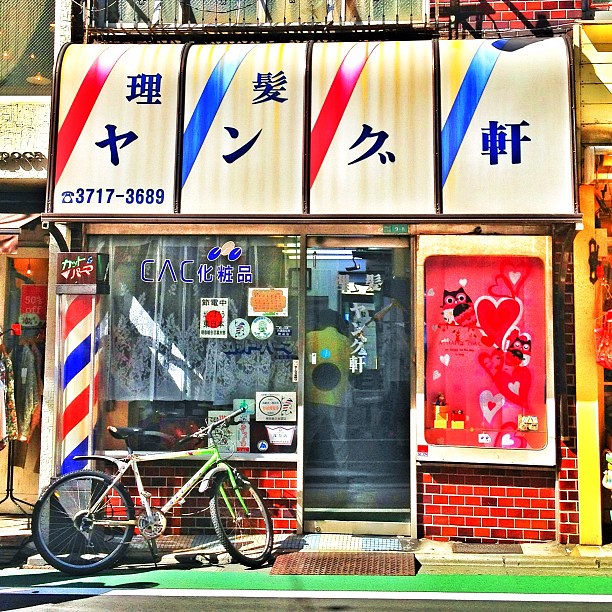This photograph depicts a vibrant storefront in an Asian country, possibly Japan or China, identifiable by the numerous Asian characters on the signage above. The building is constructed of red brick and features various fixtures that contribute to its lively appearance. Dominating the left side is a traditional red, white, and blue barber pole, hinting that this is a barbershop. A bright green and white bicycle is parked on the sidewalk near the barber pole. The storefront itself includes large windows and a glass door, through which a man and a woman can be seen inside. The right window is decorated with Valentine's-themed artwork, including hearts and an owl, while the left window displays the letters "CAC" along with a logo and several posters. Above the windows are red, white, and blue banners or awnings, and a phone number: 3717-3689, prominently displayed. A brown mat lies in front of the door, and a distinctive green stripe runs across the sidewalk in front of the shop. To the side, a yellow post marks the beginning of an adjacent store. Above the shop, a balcony or gate adds to the building's architectural interest.